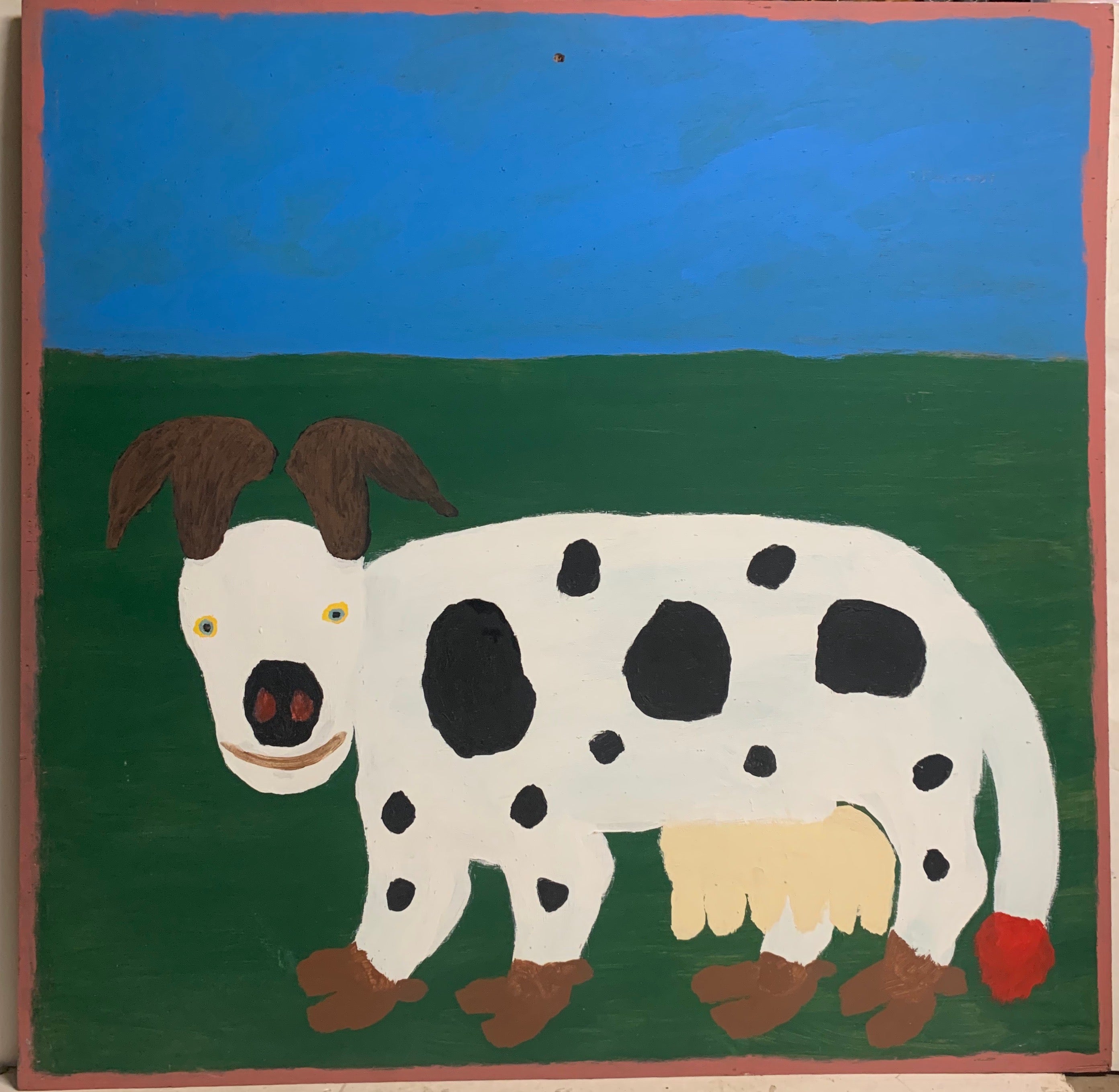The image depicts a whimsical children's painting bordered by a distinct reddish-pink line. This artwork, seemingly photographed against a gray background, features a two-tone backdrop with a blue sky occupying the top third and a greenish ground at the bottom. Dominating the foreground is a fantastical white animal, resembling a cow, with peculiar characteristics. Its body is adorned with black spots of varying sizes, and it sports small, eerie yellow and black eyes. The nose is a mix of black and red hues, complemented by a brown mouth. The creature’s legs end in brown feet, and its tail has a red tip. The udders are exaggerated with multiple nipples, painted in a yellowish-beige shade. The surreal composition and unsettling features of the animal—reminiscent of a cow with demonic attributes—add to the painting’s odd charm, capturing the uninhibited imagination typical of children's artwork.